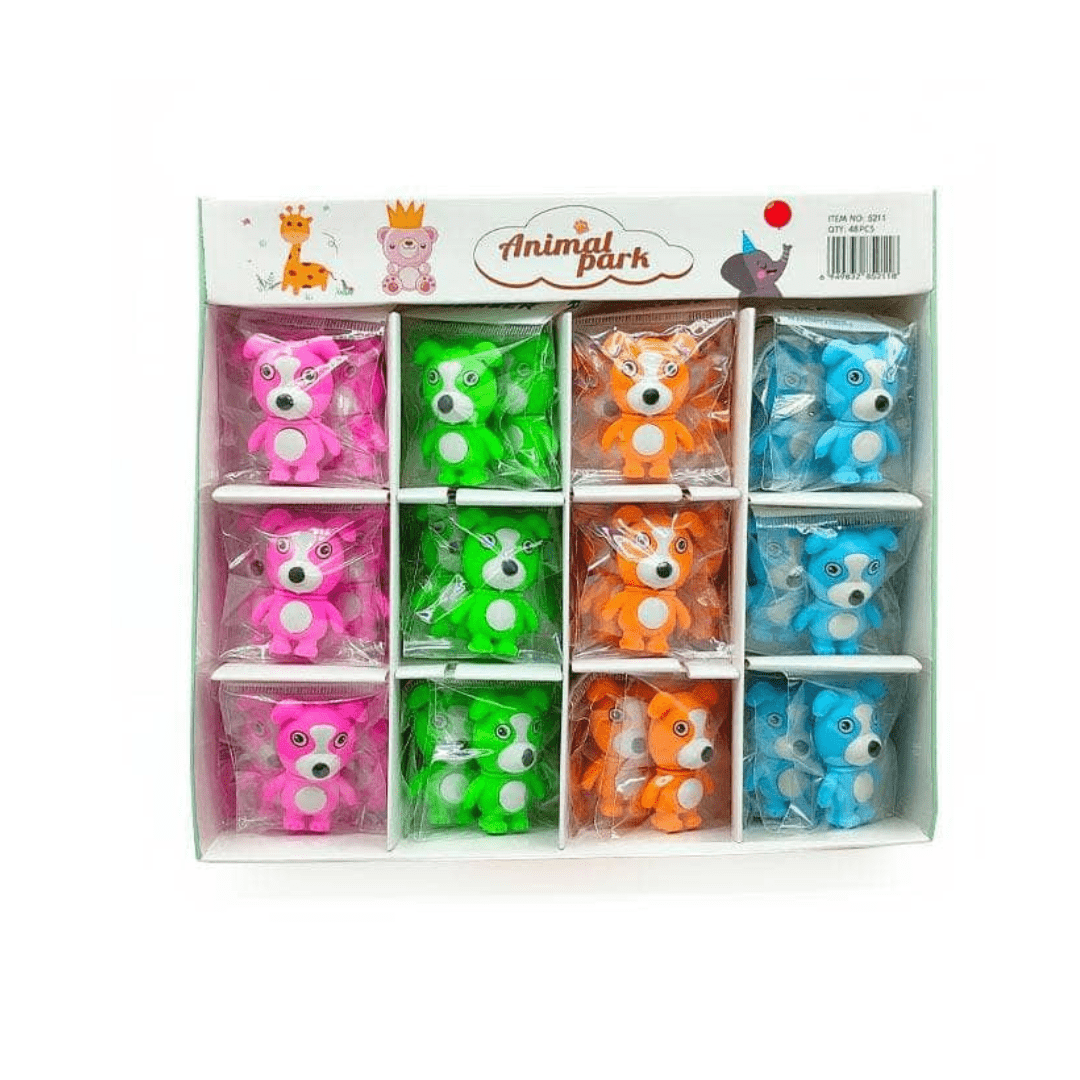This photograph showcases a colorful toy display labeled "Animal Park" at the top, with a playful illustration including a giraffe, a crown-wearing bear, and an elephant donning a birthday hat while bouncing a red balloon. The display is organized into a cardboard grid with four vertical columns and three rows of toy dogs, making a total of twelve toys. Each toy dog is individually shrink-wrapped in cellophane and stands upright, facing forward. The toy dogs come in vivid colors: hot pink, neon green, medium orange, and light blue, each featuring white bellies and white markings on their heads. The cardboard dividers create clear partitions for each toy, making the overall presentation neat and cheerful, ideal for a children's store display.